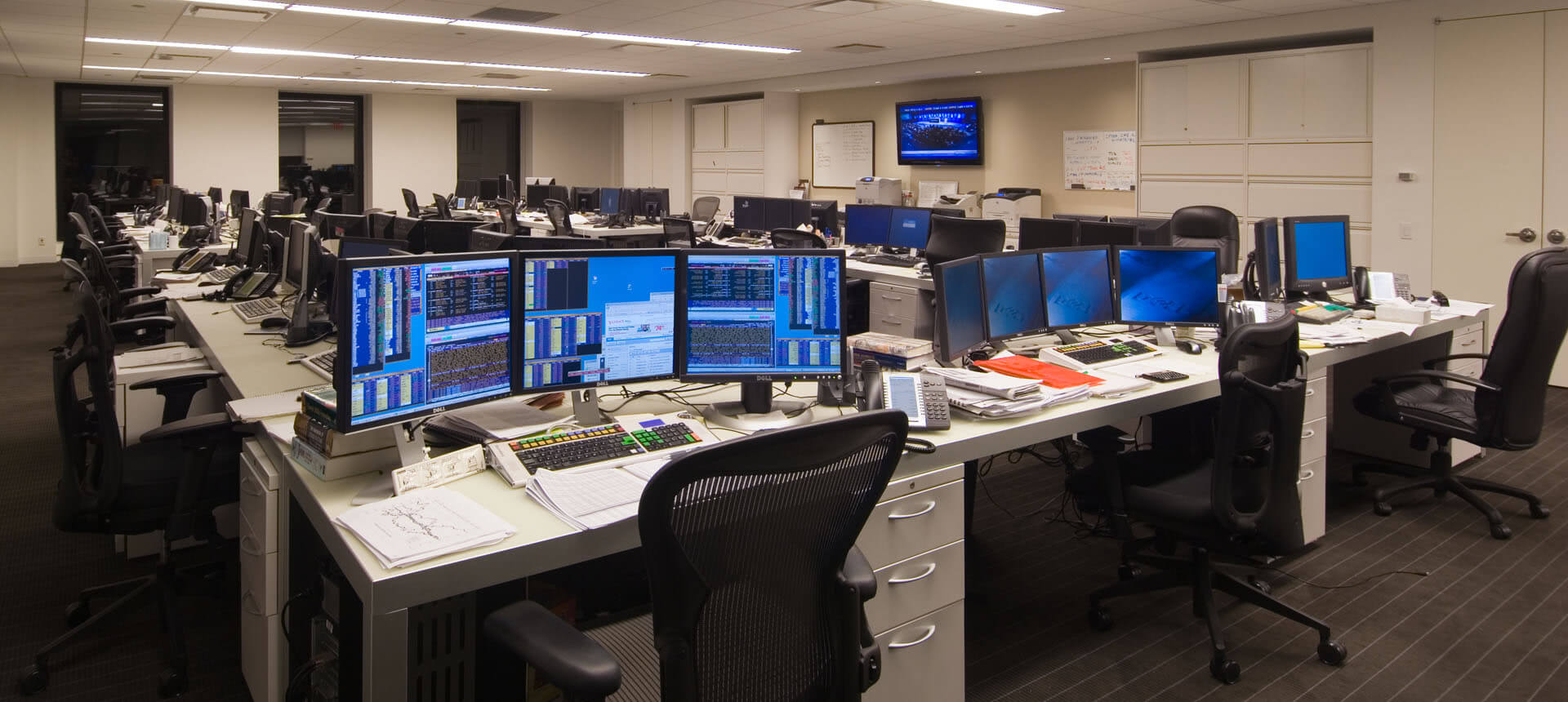This is a color photograph of an open office environment, characterized by a spacious layout without cubicles or separate office spaces. The room features numerous bunched-together desks and office chairs, all arranged in a large, brightly-lit space with white-painted walls and gray carpeting. Each desk, which is either off-white or light gray, is equipped with a varying number of computer monitors, ranging from two to four per desk, suggesting a visually intensive work setup. The desk surfaces hold keyboards and scattered papers, while shelving units and drawers with handles provide additional storage. The image foreground shows three desks with corresponding chairs, stretching back in rows throughout the sizable room. The detailed arrangement highlights a highly organized yet bustling work environment.